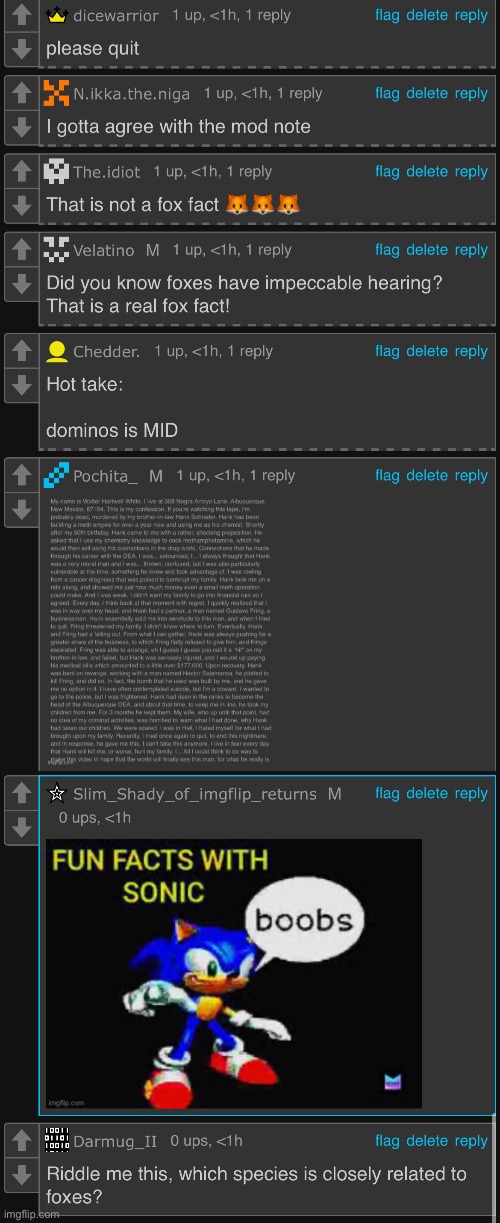The image appears to be a screenshot of a conversation in a chat group with a dark gray background and light gray text boxes. At the top, there is a user named "Dice Warrior," who has a message with one upvote, posted one hour ago with one reply. Below this, the user "N.I.K.K.A.N.I.G.A." comments with the same metadata, stating, "I gotta agree with the mod note." 

Another user, "The Idiot," responds with, "That is not a fox fact," accompanied by three fox emojis. Following this, "VelatinoM" contributes with, "Did you know foxes have impeccable hearing? That is a real fox fact," also having one upvote, posted one hour ago with one reply. User "Cheddar" then shares a "Hot Take," stating, "Domino's is M.I.D.," maintaining the same metadata.

There is a text box beneath Cheddar's comment with extremely tiny writing that becomes unreadable when zoomed in. Below this, "Slim Shady of ImageFlipReturns" posts, receiving zero upvotes one hour ago and featuring an emoji of Sonic the Hedgehog from the video game series with the statement, "Fun Facts with Sonic." The content of his blurb humorously says, "Boobs."

The final message is from "Darmug," with zero upvotes an hour ago, asking, "Riddle me this, which species is closely related to foxes?" It appears that this chat group focuses on sharing facts and discussing topics related to foxes.